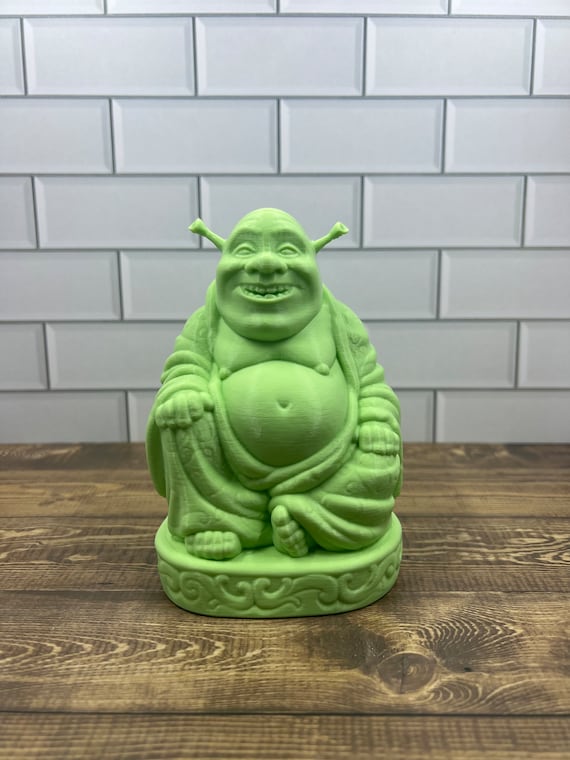This detailed photograph captures a statue of a fantasy character resembling Shrek, though it could also be interpreted as an ogre or an orc. The statue is rich in detail, prominently featuring long, black ears protruding from both sides of its head, large eyes, and wide, arcing eyebrows. It has a very wide nose with well-spaced nostrils and sparse, wide teeth. The character, with its light green color, sports a large belly and is adorned in a baggy robe that drapes over its legs, revealing its toes poking out from beneath. The figure sits atop a green base decorated with wave-like shapes, positioned on a wooden plank floor that showcases various natural shades of brown. This setting is well-lit by natural light, highlighting the wooden table with its visible grain. Behind the statue, a white brick wall, appearing gray in the photograph, provides a contrasting backdrop to the scene.